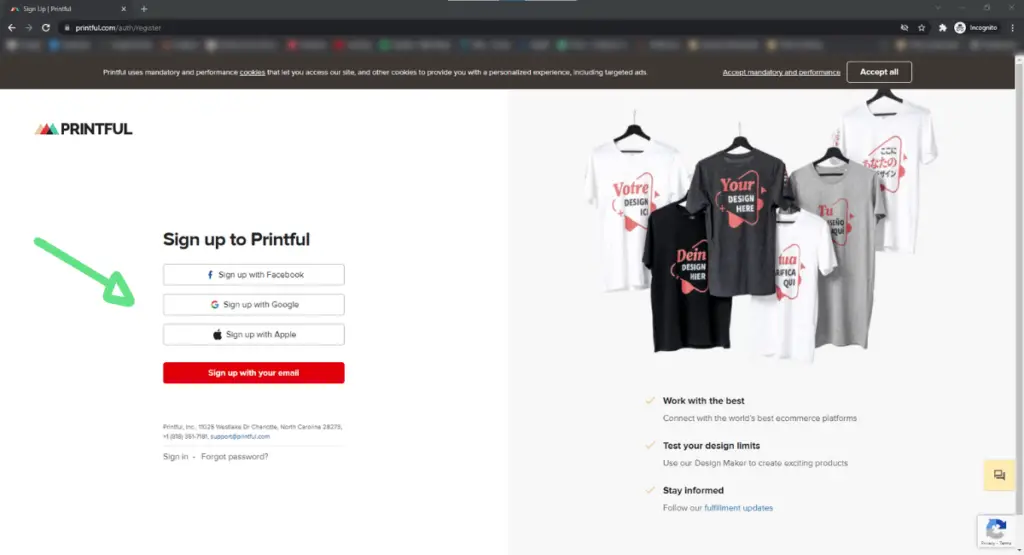This is a detailed screenshot from the Printful website captured on a dark mode Safari browser in incognito mode. The top portion of the desktop screen, including any favorited tabs or bookmarks, is intentionally blurred out for privacy. At the center of the screenshot is a prominent green arrow pointing to the signup options for Printful. The arrow specifically highlights the option to sign up with Google. Other signup options include Facebook, Apple, and email.

On the right side of the screen, six T-shirts are displayed at varying heights, each bearing the text "Your Design Here." This visual indicates that users can personalize and upload their own designs to be printed on the shirts. Below the T-shirt display, three bullet points succinctly explain Printful’s involvement in the design process and highlight the reasons why Printful is the preferred choice for custom apparel.